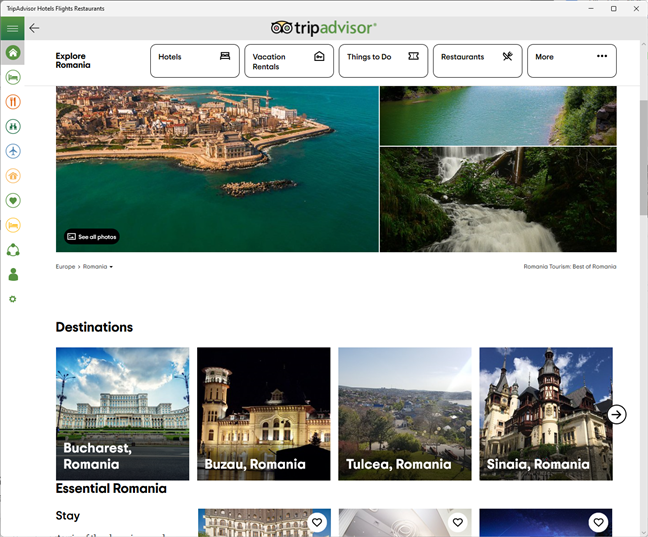This image captures the layout of the TripAdvisor home page in detail. At the very top is a thin, light gray border, approximately half an inch wide, featuring black text on the left corner that reads “TripAdvisor Hotel, Flights, Restaurants.” To the right, various icons include an X, a small square, and a dash. Directly below, a slightly darker gray, thicker border spans the width of the page. On the left, a green square is visible with three horizontal white lines. Adjacent to it is a black arrow pointing left.

Centered on this border is the TripAdvisor logo, with "Trip" in black and "Advisor" in green. Beneath the green square, there are eleven clickable icons that provide information on different categories. To their right, a black text reads “Exploring Romania.” Below this section, five white tabs with black text are stationed across another black border, offering categories such as hotels, restaurants, and things to do.

The main body of the page features a large image of a city that stretches from the top left to an inch from the right. The bottom portion of this image showcases a vibrant blue body of water. To the right of this image, two smaller, equally divided pictures are displayed. The top picture shows a river bordered by grass, while the bottom image captures a waterfall flowing down the middle, surrounded by lush greenery and possibly wheat or trees.

Further down on the left side, bold black text reads “Destinations,” accompanied by four more images of various landmarks in Romania, each labeled with white text indicating the location. Underneath these images, the section titled "Essential Romania" features additional categories. The "Stay" section is partially visible, showing the top edges of three more images.